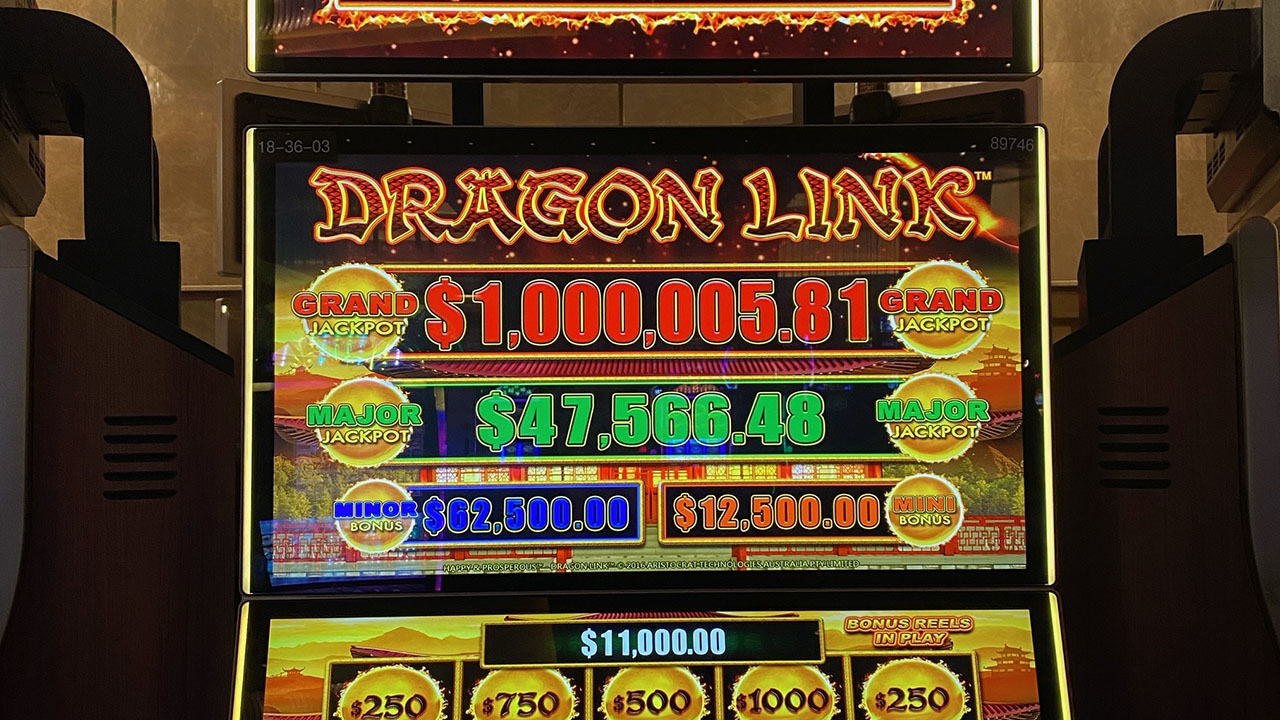This photograph features the upper portion of a slot machine, prominently displaying the game title "Dragon Link" in red text with a golden outline, styled with an Asian-inspired font. At the top, the Grand Jackpot is highlighted, indicating a prize of $1,000,005.81. Below, the Major Jackpot is shown as $47,566.48. Further down, the Minor Bonus lists a value of $62,500, despite being unusually higher than the Major Jackpot. Next, the Mini Bonus displays an amount of $12,500. Additionally, the bonus reels in play are noted next to a figure of $11,000. The screen showcases vibrant colors, including reds, greens, blues, golds, yellows, oranges, and purples, adding to the visual appeal. The bottom section features potential win amounts displayed as $250, $750, $500, $1,000, and $250 from left to right. The background is blurred, hinting at the presence of adjacent machines. The photo captures the concentrated and colorful essence of a bustling arcade environment.